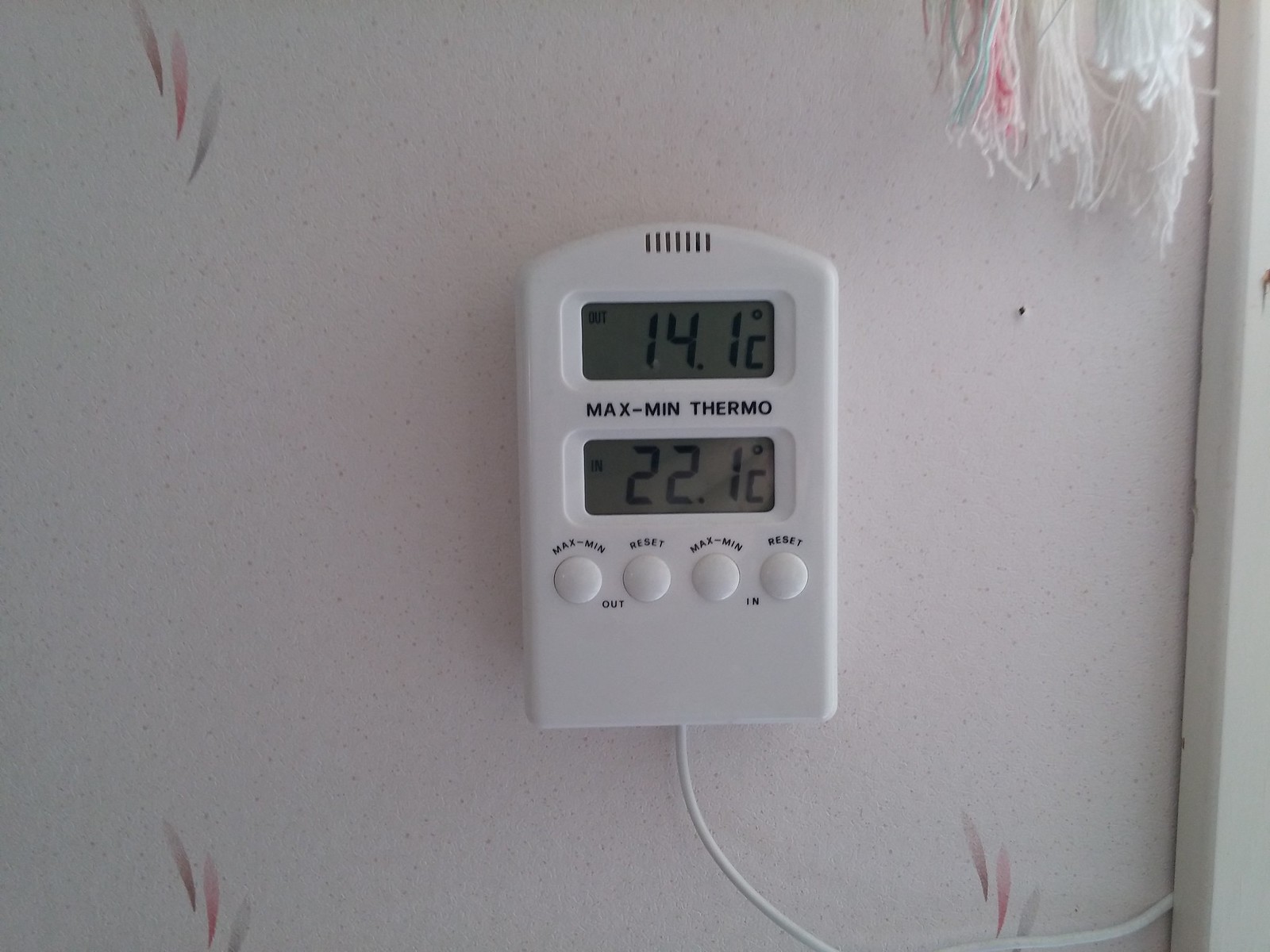This photograph captures an indoor scene set within a room with white walls adorned with a few paintings. In the top right corner, a pattern of horizontal lines in brown, red, and gray is visible, repeating in smaller segments near the bottom and right side of the picture. 

Hanging from the top right of the frame are strands that appear to be parts of a blanket, featuring predominantly white strings with hints of blue and pink interwoven. A white post is situated on the right, from which a white cord extends. This cord connects to a white thermostat mounted on the wall. 

The thermostat is detailed with small black lines at the top, and its screen displays "OUT" along with a temperature of 14.1°C. Below this, it reads "Max Min Thermo" and shows another temperature of 22.1°C. There are several buttons labeled "Max Min Reset" beneath the screen.